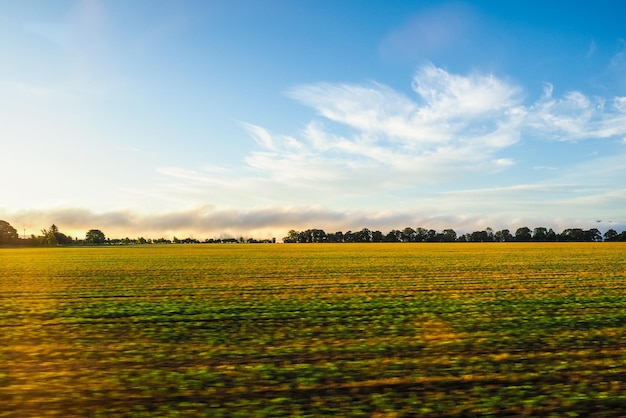The image depicts an expansive farmer's field with neatly trimmed grass and rows of small green and yellow crops, extending across the foreground. In the background, a line of tall, lush green trees frames the horizon, standing beneath a beautifully varied blue sky. Puffy white clouds, some slightly darker near the base, dot the sky from left to right, creating a picturesque backdrop. Evident sunlight casts an angled yellowish light, suggesting either sunrise or sunset, adding a warm glow to the serene and wide-open farmland. The photograph, taken on a clear day, captures the tranquil, pleasant essence of rural life, splitting its composition evenly between the cultivated rows of the lower half and the vibrant sky above.